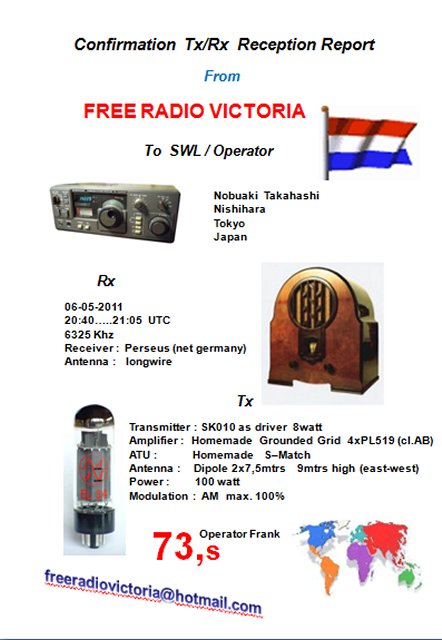The image appears to be a confirmation of a transmission and reception report from Free Radio Victoria to an SWL (Shortwave Listener) operator. Set against a white poster, the top of the image prominently displays "Confirmation TX/RX Reception Report" in black text. Below that, "From Free Radio Victoria" is highlighted in red, blue, and black. To the right, a flag with horizontal red, white, and blue stripes -- distinct from the American flag -- is shown.

Beneath this, on the left side of the image, is an illustration of a shortwave radio, accompanied by the text "Nobuaki Takahashi, Nishihara, Tokyo, Japan." The section labeled "RX" details the reception: "06-05-2011, 20:40-21:05 UTC, 6325 kilohertz," "Receiver: Perseus, NET Germany," and "Antenna: Long Wire." This is adjacent to another image of a vintage radio device, resembling a 1920s tabletop model.

Further down, the section labeled "TX" refers to the transmitter, specifying details such as "Transmitter: SK010S driver 8 watts amplifier," "Homemade grounded grid 4XPL519 (CLAV)," "ATU: Homemade S-MATCH," "Antenna: Dipole 2x7.5 meters, 9 meters high east-west," "Power: 100 watts," and "Modulation: AM, max 100%." Additionally, there's an image depicting a cylindrical component, likely a glass vacuum tube.

A global map in the lower-right corner highlights various continents and countries in distinct colors: Asia in red, Africa in purple, South America in orange, Australia in green, and the United States and Canada in blue. Beside it is the text "Operator: Frank, 73s."

At the bottom of the poster, in blue print, the email address "freeradiovictoria@hotmail.com" is provided for contact.